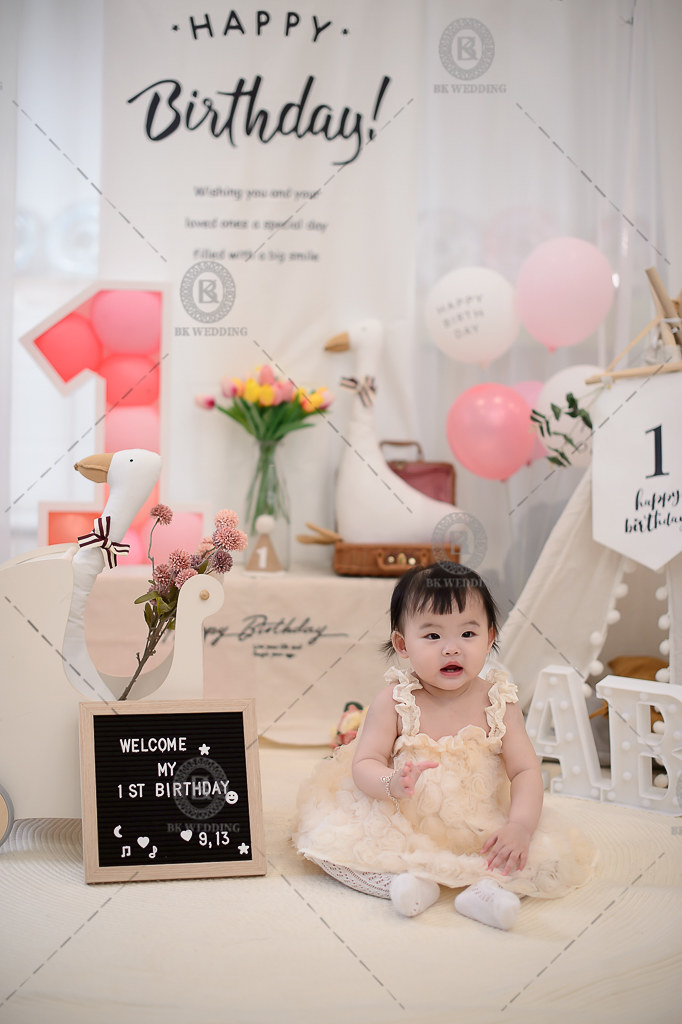The photograph captures the heartwarming moment of a young Asian girl celebrating her first birthday. She is seated cross-legged on a white floor at the bottom right of the image, wearing a light pink dress with white socks. Her dark brown or black hair is adorned with adorable bangs across her forehead. With a charming smile and a little hand raised, seemingly waving to her mommy or daddy, she exudes joy and innocence. Around her wrist is a delicate bracelet.

To the left of the girl is a small black chalkboard with a wooden border, displaying the message, "Welcome, my first birthday," and the date, "9-13" — indicating September 2013. The backdrop is a meticulously staged setting featuring an array of colorful balloons in shades of white, pink, light pink, and gray. Directly behind her, a large pink number "1" stands prominently beside a bouquet of flowers.

Stuffed animals resembling swans or geese are scattered amidst bits of furniture in the background, enhancing the festive ambiance. A vertical banner with the words, "Happy Birthday," arcs above her in bold black script, adding to the celebratory atmosphere. The image is exquisitely detailed, capturing the essence of a joyful milestone in the child's life, preserved as a beautiful memory in photographic realism. Additionally, faint photographer’s markings suggest it might be a proof sent for parental approval before finalization.